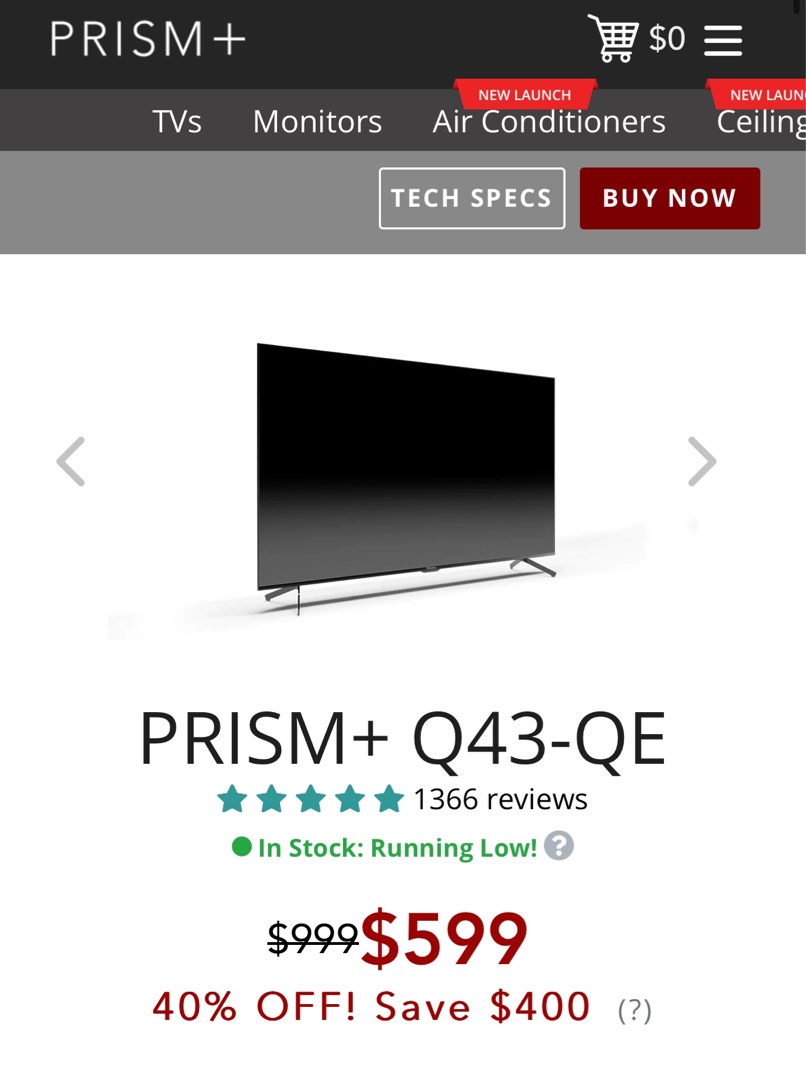The website screenshot appears to be from the PRISM Plus official site. The topmost section features a black navigation bar displaying the PRISM Plus logo on the left and a shopping cart icon showing $0 on the right, alongside a hamburger menu represented by three horizontal lines.

Below this, there's a secondary gray bar with white text listing product categories: TVs, monitors, air conditioners, and ceilings. Notably, "air conditioners" and "ceilings" are accompanied by a "New Launch" banner in red with white lettering.

Further down, another gray bar contains two interactive buttons. The first button labeled "Tech Specs" is gray, while the second, labeled "Buy Now," is red with white text.

Dominating the middle of the page is a visual display of a TV model, the PRISM Plus Q43QE. Flanking the TV image are navigation arrows for browsing additional images. Below the TV image, the model name is prominently displayed along with a 5-star rating based on 1,366 reviews. A status indicator shows "In Stock" but notes it is "Running Low" in green text, accompanied by a gray circle with a white question mark for additional information.

The listed price for the TV is shown as $999, which is crossed out and replaced by a discounted price of $599 in red text, boasting a 40% reduction and a $400 savings. The color scheme of the website is predominantly black, gray, red, and white, with the star ratings highlighted in a turquoise color.